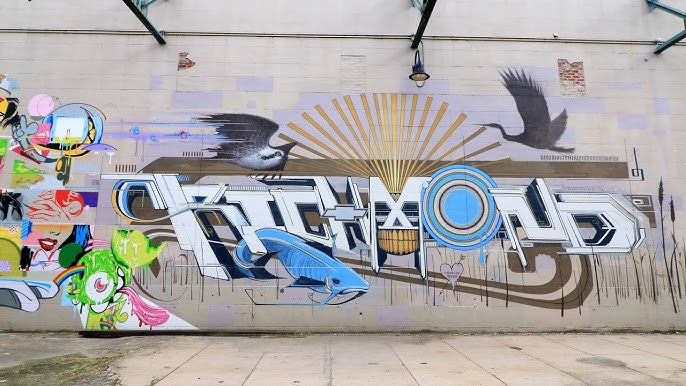The photograph captures an outdoor scene featuring an old, stained sidewalk in the foreground with a patch of grass or weeds in the lower left corner. The sidewalk is a light grayish-brown color with darker gray spots scattered around. Behind the sidewalk stands an aged cement wall, colored a light grayish-tan, adorned with various pieces of artwork. 

The artwork in the center includes large, white block letters that are stacked and curved, making them difficult to read. Emerging from one of these letters is a blue fish, positioned so that both its front and right side are visible. Surrounding the central letters is an alternating blue and gold pattern forming an 'O'. Above this, a couple of black birds are depicted in flight.

On the left side of the mural, there are smaller, colorful images. These include the lower half of a woman's face featuring bright red lipstick and what looks like a sunburst in a yellowish-tan hue. The wall is sectioned by several black bars across the top, each appearing to support lanterns.

The array of colors in the mural includes light blue, white, violet, black, green, yellow, beige, tan, and gold. The photograph appears to be taken from about 15 to 20 feet away, suggesting a viewpoint from across the street, directly facing the graffiti. Above the mural, beams are visible with lights hanging from them, while the ground below shows signs of age with wet or dirt spots. The exact time of day or whether the photo was taken indoors or outdoors cannot be determined from the image.